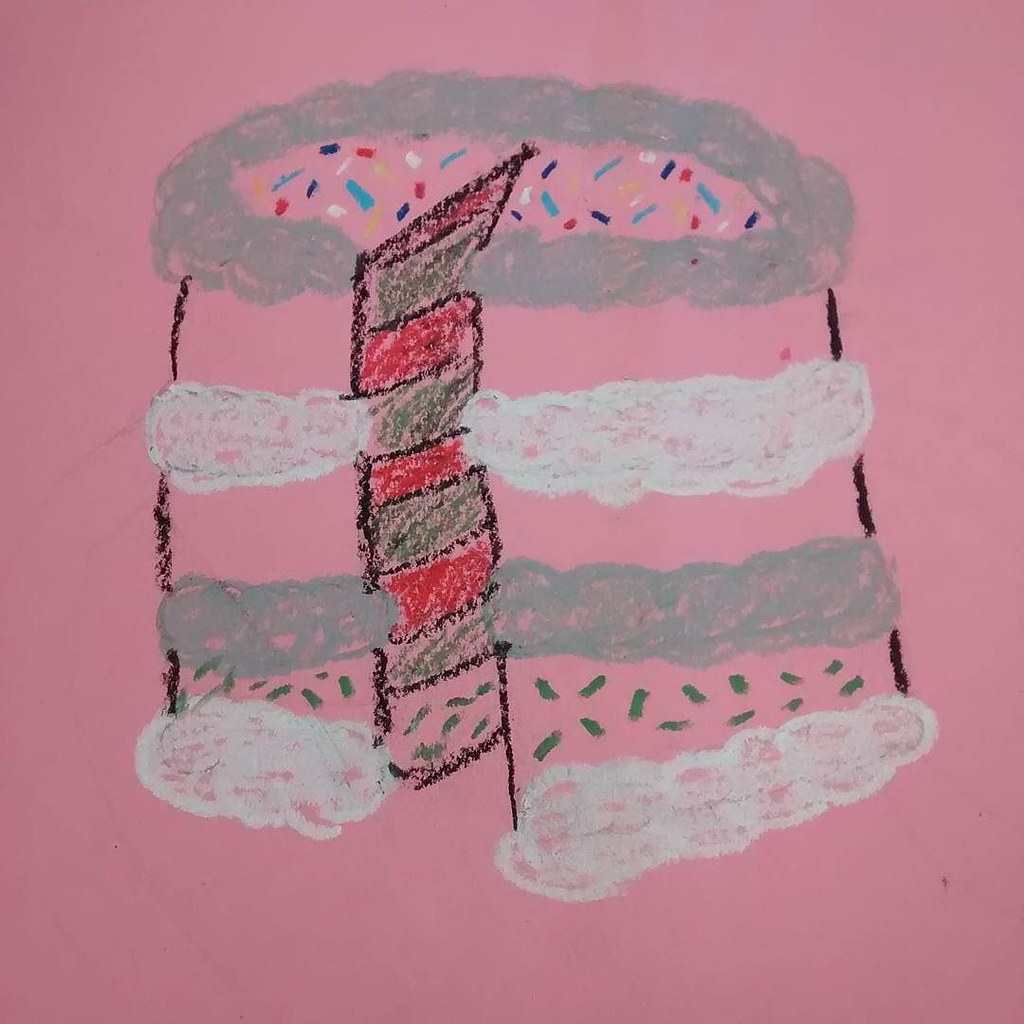This charming and whimsical drawing, likely created by a child, features a delightful birthday cake set against a vibrant pink background. The cake's outer design cleverly incorporates the pink from the background, making it appear vividly integrated with its surroundings. At the base of the cake, a gray circle forms a foundation with a playful arrangement of looped circles representing the icing.

The cake itself is decorated in a layered pattern alternating between the vibrant pink of the background and hues of gray and white, giving it a festive, multi-tiered appearance. These layers appear in the following sequence: starting with gray icing loops, followed by a pink space, then white icing loops, another pink space, gray icing loops, a final pink space, and ending with white icing loops.

Inside the cake, the artist has illustrated intricate layers filled with green, interwoven with streaks of black and red, adding depth and richness to the design. The cake is sprinkled with a delightful array of colorful dots in blue, green, white, and black, scattered generously across the surface. Green dots are also meticulously placed throughout the bottom layer, providing a cohesive and joyous visual treat.